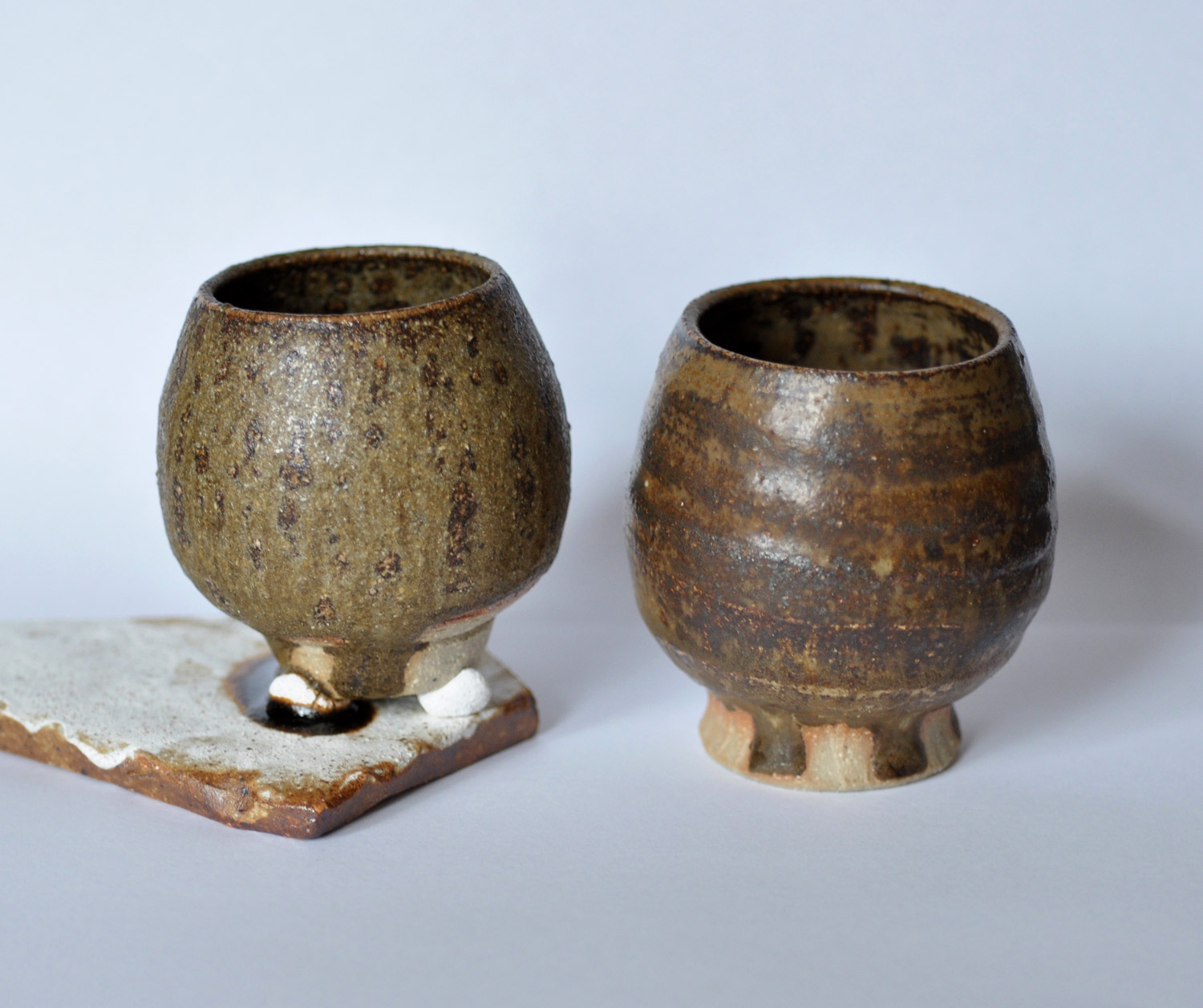The image features two ancient, rustic-looking ceramic cups against a stark white background. Both cups showcase signs of aging and wear, giving them a distinctly vintage feel. The cup on the left, which could be described as a chalice, has a greenish-brown hue with a freckled pattern and stands on a unique base that resembles small white marshmallows resting on a thin brown stone with a white top. It is slightly uncentered towards the left side of the image. The cup on the right is a dark brown with subtle horizontal striping and a flared base composed of alternating dark and light brown squares, adding a decorative touch to its cylindrical form. Both cups are upright and seem to be functional for holding liquids, captured in high-resolution detail that highlights the texture and material imperfections accrued over time.